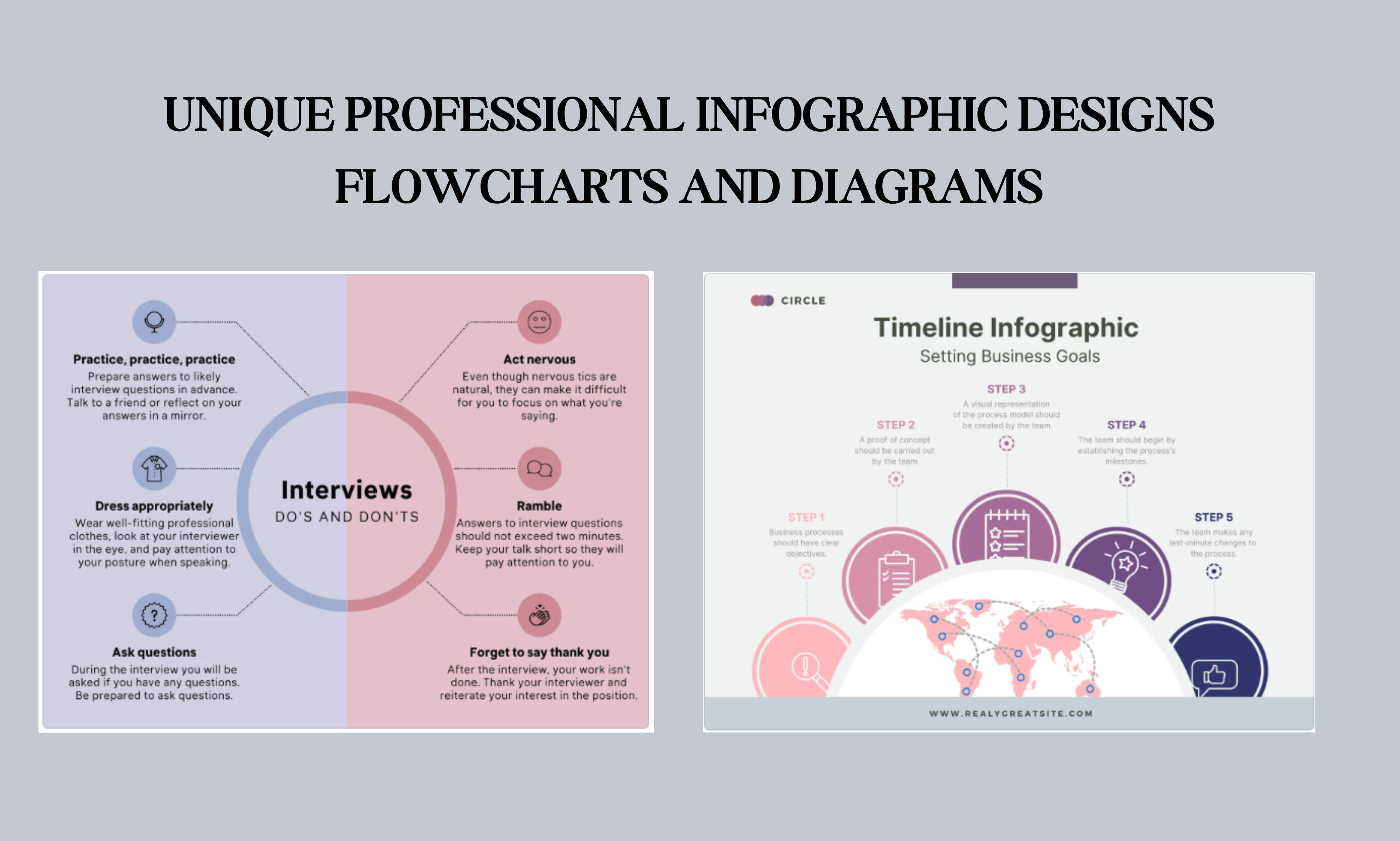The image is a horizontally rectangular, multi-color print piece with a grayish background and no borders. At the top, black text in all caps reads "UNIQUE PROFESSIONAL INFOGRAPHIC DESIGNS" followed by "Flowcharts and Diagrams." Below this text are two equally-sized illustrations, one on the left and one on the right. 

The left illustration is a detailed infographic about interview do's and don'ts, with a central circle labeled "INTERVIEWS" and "Do's and Don'ts" in smaller text beneath. The left half of the circle features three blue blowout points: "Practice," "Dress Appropriately," and "Ask Questions." The right half has three pink blowout points: "Don't Act Nervous," "Don't Ramble," and "Don't Forget to Say Thank You." 

The right illustration is a timeline infographic with a white background, focusing on "SETTING BUSINESS GOALS." It steps through stages one to five, which, though too small to read in detail, are marked above a semicircular globe illustration. This globe highlights all countries in shades transitioning from pink to dark purple and navy. The entire design creatively blends color illustrations with informative text.